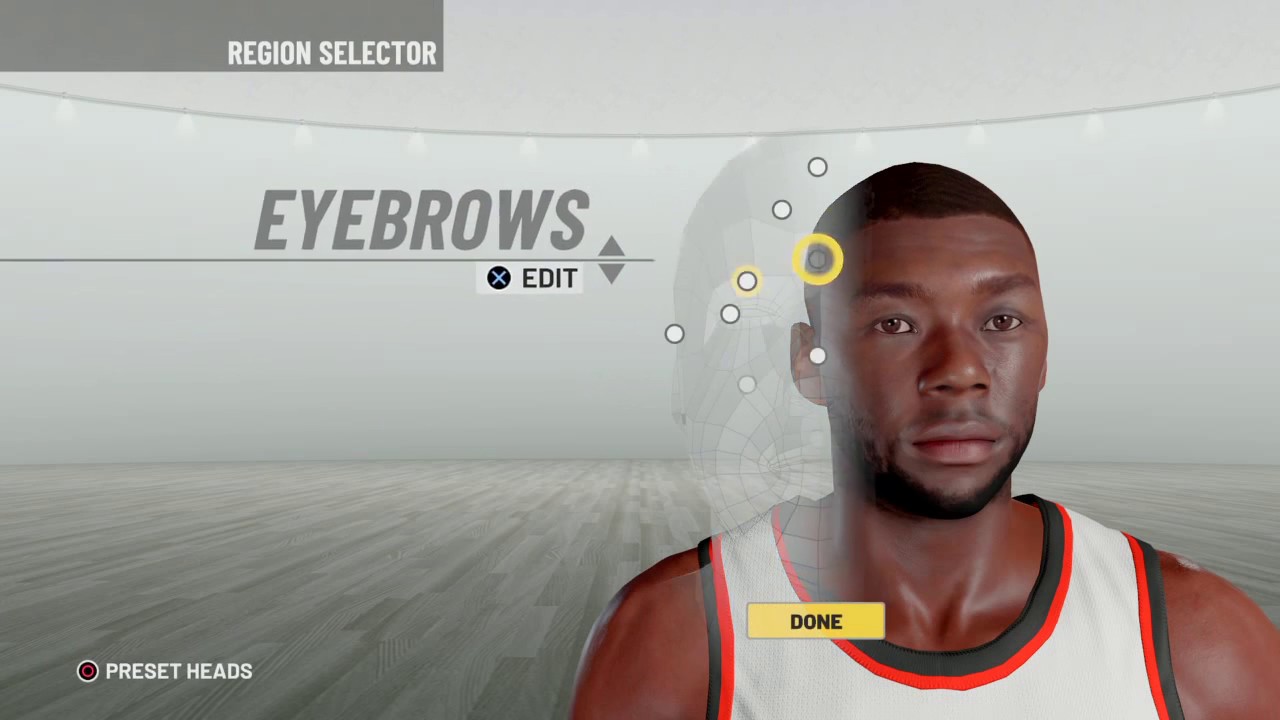This is a detailed screenshot of a video game character editor. The background features gray walls and a gray wooden floor, providing a neutral backdrop for the editing interface. 

In the upper left corner, there's a gray rectangle with the label "Region Selector" in white font. Directly below this, a black line divides the text. On this line, the word "Eyebrows" is prominently displayed in large gray font. Below this, an up arrow and a down arrow in gray allow for adjustments. Below the line, there's a small white rectangle housing a black circle with a white 'X'. To the right of this, "Edit" is written in black font.

In the lower left corner, there is a white circle with a black circle inside, which has a red circle at its center. To the right of this symbol, "Preset Heads" is written in white font.

On the right side of the image, a virtual character is displayed. The character is a Black man wearing a white basketball jersey outlined with black and orange trim. He has short black hair and his skin has a shiny appearance. Facing forward, his expression is neutral, neither smiling nor frowning. Multiple white circles are arranged around his head, likely indicating adjustable features. 

To the left of the character and on his neck, there is a yellow button labeled "Done" in black font, signaling the option to finalize changes.